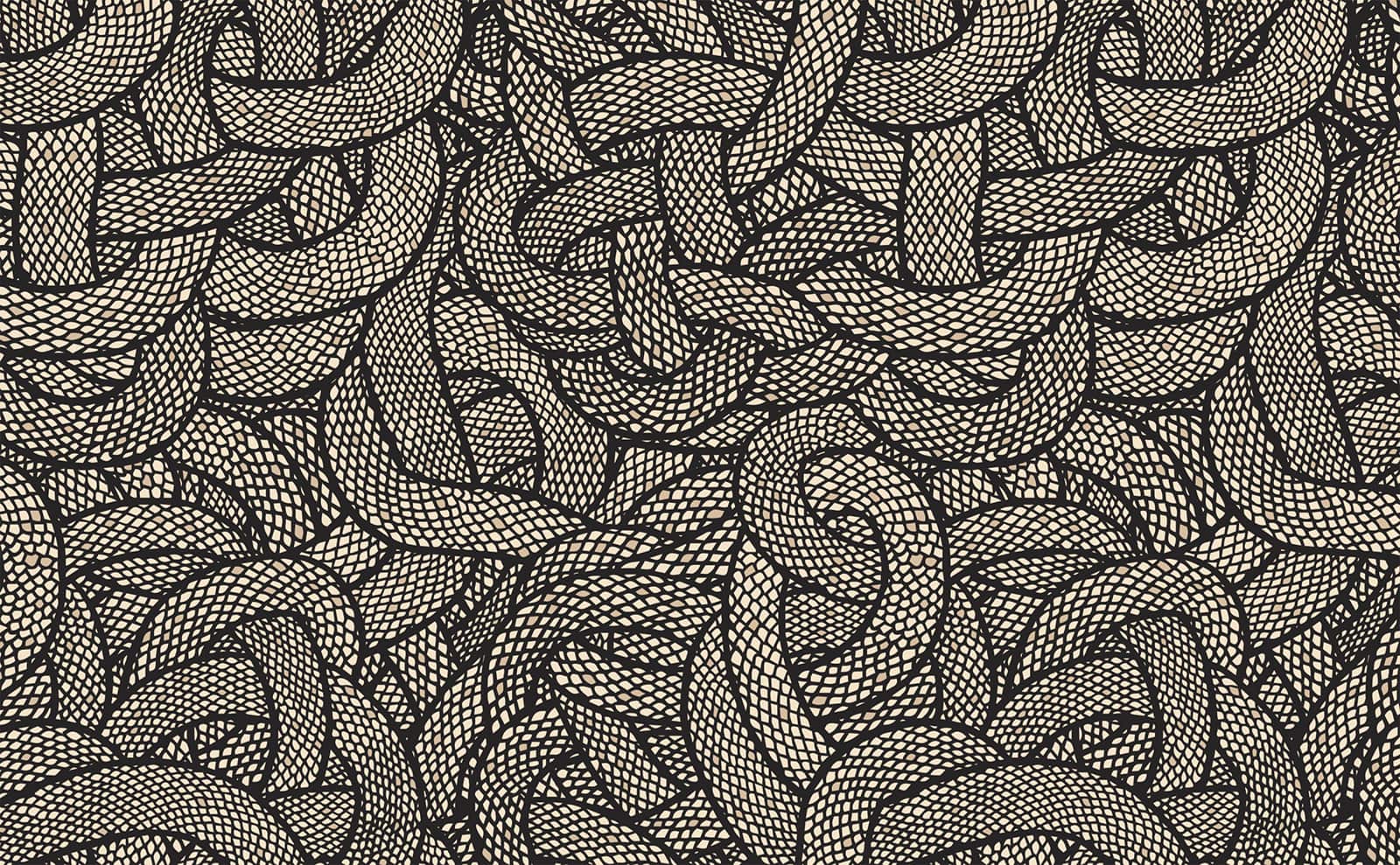The image is a rectangular illustration, longer horizontally than vertically, featuring a complex and intertwined arrangement of coils that resemble strings or ropes with a snakeskin pattern. The coils have prominent black outlines and are adorned with scales mostly in white and gray, with sporadic light brown or beige scales adding depth to the texture. The twisty and turny layout of the coils creates a series of knots, curves, and loops, giving the impression of an intricate and tangled mass of scaled ropes. The entire sketch is framed by a black border, enhancing the detailed and serpentine-like design of the coils within.